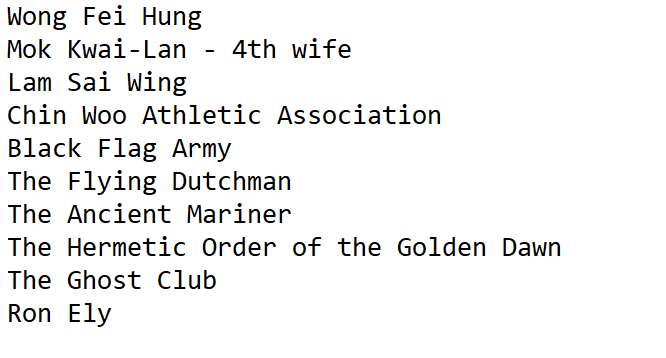The image displays a simple, unbordered white sheet with black text, likely styled in an OCR or Courier font. Arranged in a vertical list, each of the ten lines is fully capitalized. The names and titles, resembling a family tree, list, or catalog, include: WONG FEI HUNG, MAK KWAI LAN, FOURTH WIFE, LAM SAI WING, CHIN WOO ATHLETIC ASSOCIATION, BLACK FLAG ARMY, THE FLYING DUTCHMAN, THE ANCIENT MARINER, THE HERMETIC ORDER OF THE GOLDEN DAWN, THE GHOST CLUB, and RON ELY. Each entry appears in large, bold text, creating a stark contrast against the white background.